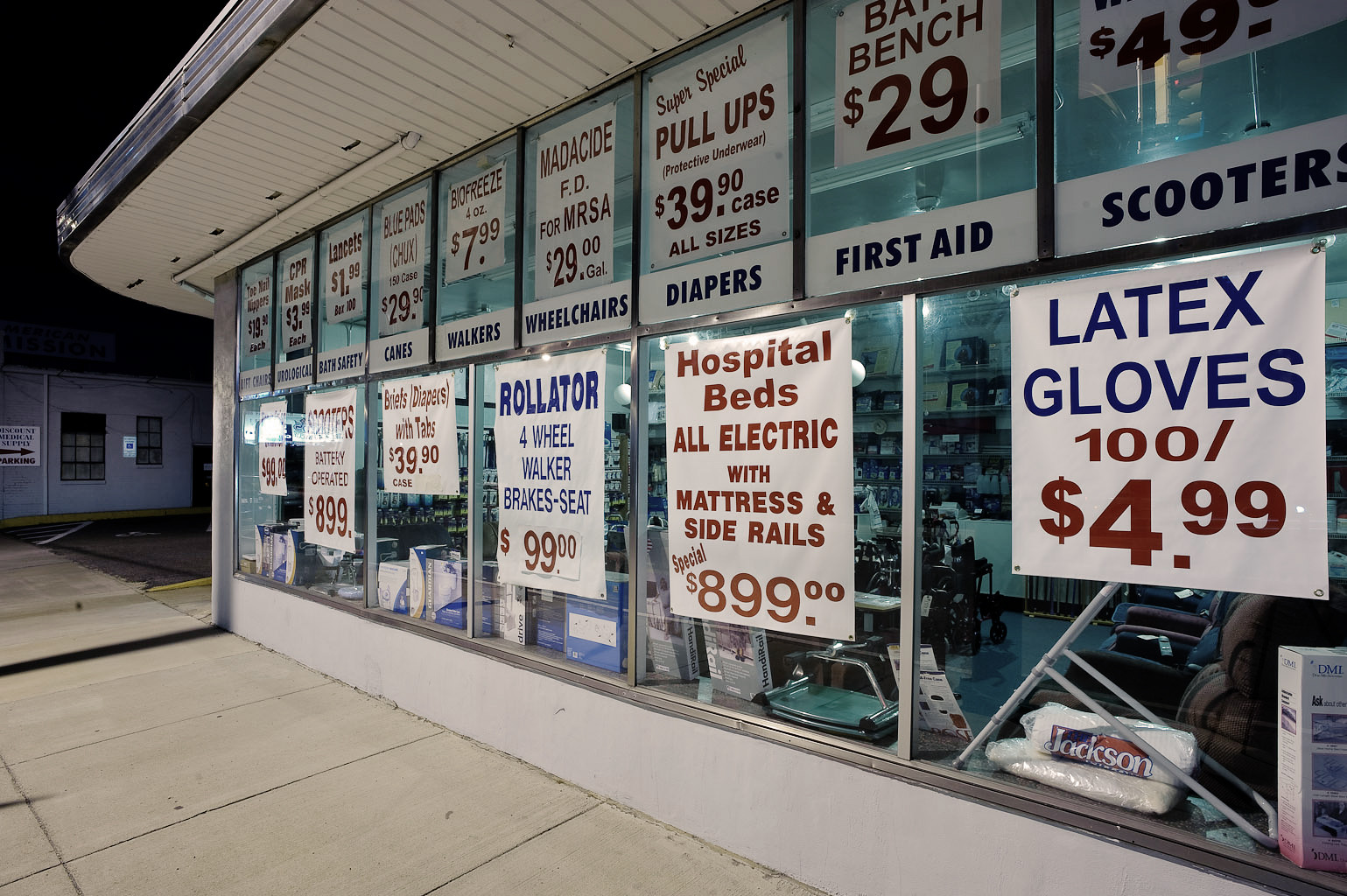The image captures a nighttime scene of a storefront likely specializing in assisted living products. The sky is pitch black, indicating evening hours. Adjacent to the store, a receiving dock possibly belonging to another business is partially visible. The store's windows are plastered with various signs advertising an array of products essential for assisted living. Prominent items include canes, walkers, wheelchairs, diapers, first aid supplies, and scooters.

Detailed product advertisements feature bleach, pull-up diapers for $39.90 per case, MRSA-targeted gel for $29, and latex gloves priced at $4.99 per 100 units. The signage primarily employs red text for highlighting sales, while blue text describes the products.

Peering through the windows reveals a glimpse inside the store, showcasing items such as pillows, stools, and couches. The overall aesthetic, including the pricing and font styles, hints that the photo might originate from the 1960s or 1970s. Every window is adorned with advertisements, including a noteworthy rollator walker with brake seats priced at $99. The prices starkly contrast with what one would expect in today's economy, underscoring a bygone era.